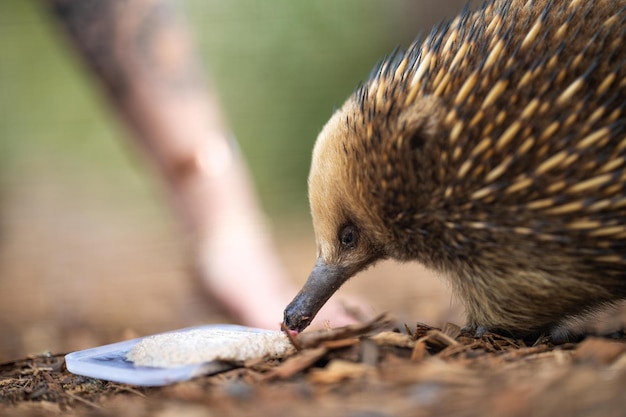In this outdoor setting, the focus is on a small, brown, spiked animal that resembles an echidna, with elements suggesting it could be similar to a porcupine or hedgehog. The creature's spiky body features a mix of brown, beige, and black quills. Its long, slender snout is dark brown and it is seen sniffing or licking something on the dirt ground, which appears to be a discarded plastic lid containing a white, creamy substance, possibly resembling runny oatmeal or grits. The blurred background shows wood chips and part of a human's tattooed and watch-wearing arm, adding context to the scene. The rest of the image, except for the central animal subject, is out of focus, drawing attention to the echidna-like animal's curious behavior.